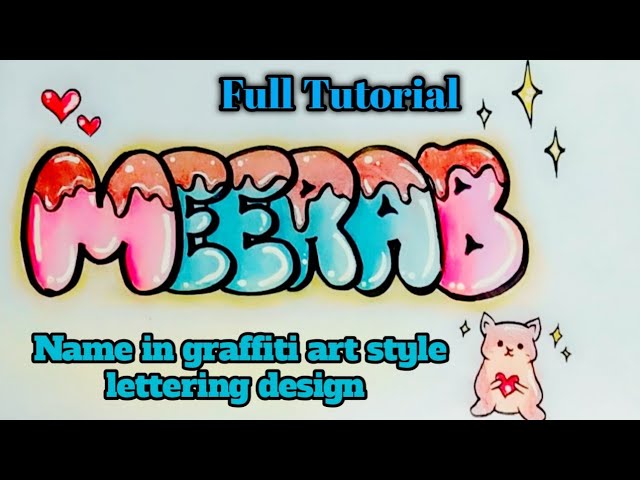This image appears to be a thumbnail or screenshot from a YouTube video or presentation slide. It features a white backdrop framed by black borders on the top and bottom. At the top of the image, blue lettering with black shadows reads, "Full Tutorial." Below that, in a whimsical, syrup-drizzled graffiti style, the name "MEERAB" is displayed. The "M" and the "B" are rendered in pink, while the rest of the letters are in blue, all with a brown drizzle effect resembling syrup. Above the "M," two small hearts are drawn, and around the "B," several diamond-shaped sparkle effects are visible. Beneath the name, more blue lettering with a black outline reads, "Name in Graffiti Art Style Lettering Design." To the right of this text, there is a cute, chibi-style creature with a cat-like head and a round body, holding a heart, colored mostly in pink. Sparkles surround this adorable character, enhancing the playful and artistic theme of the image.